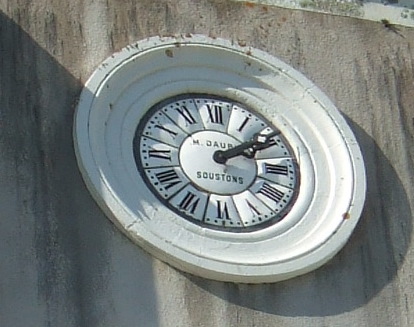This image depicts a distinctive antique clock, prominently centered on a stained, possibly outdoor concrete wall. The clock features a large, round design reminiscent of a hubcap, characterized by a wide, raised outer border and multiple circular rings leading inward. Painted white, the clock exhibits some rusting at the top, lending it a vintage charm. The clock face, adorned with black Roman numerals, is encircled by a black band and features black minute and hour hands, indicating the time as ten after two. Within the inner circle, the names "M DAUB" and "S O U S T O N S" are inscribed above and below the hands, respectively. Shadows cast by the clock create a rounded shape on the bottom right and a distinct shadow on the left side, further accentuating its dimensionality.